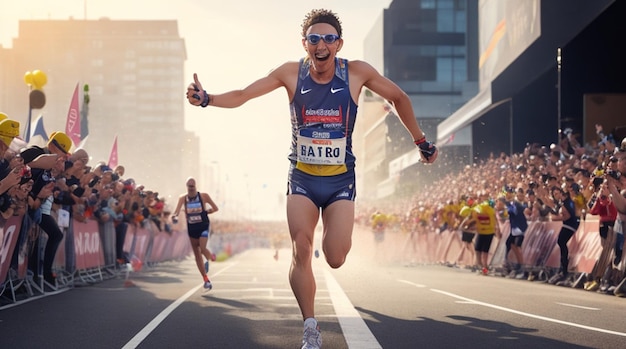The image captures the jubilant moment of a city race, highlighting the clear winner—a young man named Batro, as indicated by the paper attached to his blue Nike racing outfit. With an enthusiastic smile and a thumbs up directed at the camera, Batro exudes excitement as he crosses the finish line. His short, curly brown hair and the goggles he wears add to his distinctive appearance, along with his blue shorts, white tennis shoes, and a glove on his left hand. The second-place runner is visible but blurry and significantly farther behind, emphasizing Batro's lead. The race takes place on a paved street marked with white lines, surrounded by tall urban office buildings and residential structures. Spectators line both sides of the street, cheering fervently, with arms raised, confetti in the air, and mobile phones capturing the moment. Sponsor stands and balloons indicate the race's popularity and festive atmosphere. The bright daylight and bustling cityscape further augment the energy and setting of this thrilling race event.